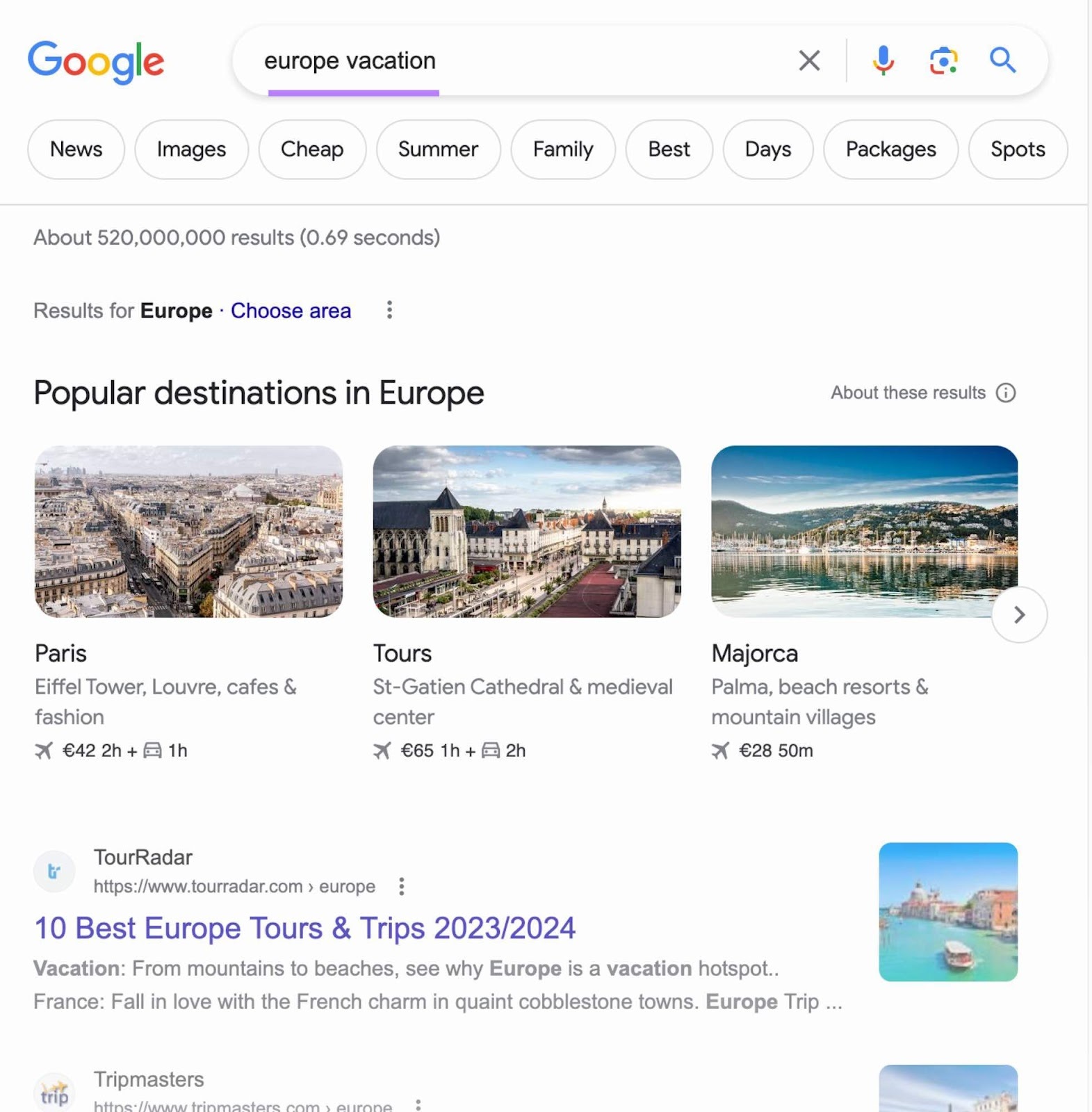The image is a screen capture of a Google search results page for the query "Europe vacation." The search bar prominently displays "Europe vacation" as the input text. Below the search bar, the results begin with a section titled "Popular destinations in Europe," featuring individual listings for Paris, Tours, and Majorca, each accompanied by a representative thumbnail image—Paris with an iconic city view, Tours with a scenic depiction, and Majorca with a picturesque waterfront scene.

Following this, a listing from the site "TourRadar" appears, offering a link titled "10 Best Europe Tours and Trips 2023/2024." Adjacent to this link is a small thumbnail image related to the content of the site.

Further down, another result from the site "TripMasters" is visible, although specific details of its offerings are not provided in the caption. Surrounding these primary links are various smaller thumbnail images associated with the respective websites or the general search results. 

At the top of the results, there's an indication of the total number of search results found, approximately 520 million, suggesting that the user might want to refine their search criteria to yield more specific and manageable results.